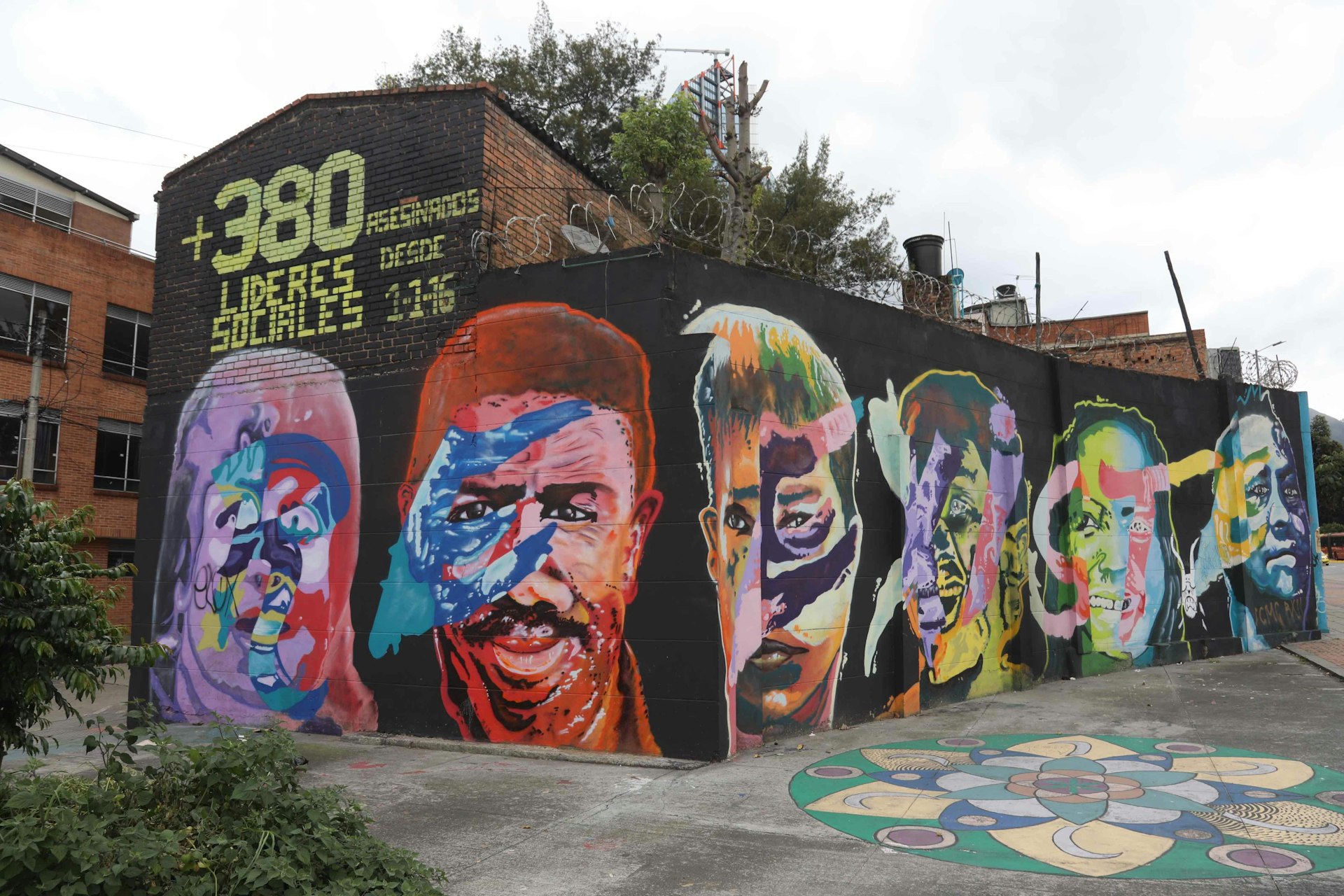This full-color, squared photograph captures an outdoor scene in natural daylight, likely taken in a non-English-speaking country given the visible text. Centered in the image is a mural on a black brick wall, featuring six graffiti-style facial portraits, each obscured by splashes of vibrant, varied colors such as red, white, purple, green, and blue. The detailed text at the top of the mural reads "PLUS 380 LIDERES SOCIALES DESDE 1-1-16." To the left of the mural is another brown brick building partially visible, while in the lower left corner of the image, there is a bush and a distinctive circular design with colorful geometric patterns, including crescent moons and flowers, painted on the ground. The background sky is overcast, and a few trees peek into the frame, enhancing the outdoor ambiance.